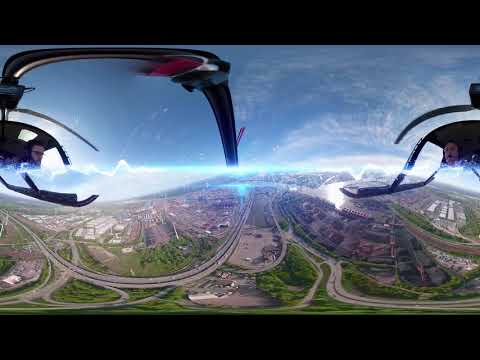The image is an aerial, 360-degree panoramic view of a very large city taken during the daytime with a slightly cloudy blue sky. The primary focus is the expansive urban landscape below, featuring a complex network of intertwining highways, streets, and numerous buildings that extend into the distance. There are green trees scattered around, adding a touch of nature to the metropolitan scene.

The image appears distorted, characteristic of a fisheye lens, making straight lines curve near the bottom of the frame. This distortion adds a dynamic, somewhat surreal quality to the photograph. The edges of the image have a black border, and within the top and bottom sections of the frame, you can see portions of the helicopter's interior, adding context to the aerial viewpoint.

On the left and right sides of the image, there are partial, distorted figures of what seem to be the helicopter's pilots, halfway cut off due to the image's curvature. From this high vantage point, features on the ground, such as streets, houses, and larger buildings—including factories or industrial zones—are visible. The far background of the image hints at a river or lake, enhancing the sense of depth and scale in the photograph.